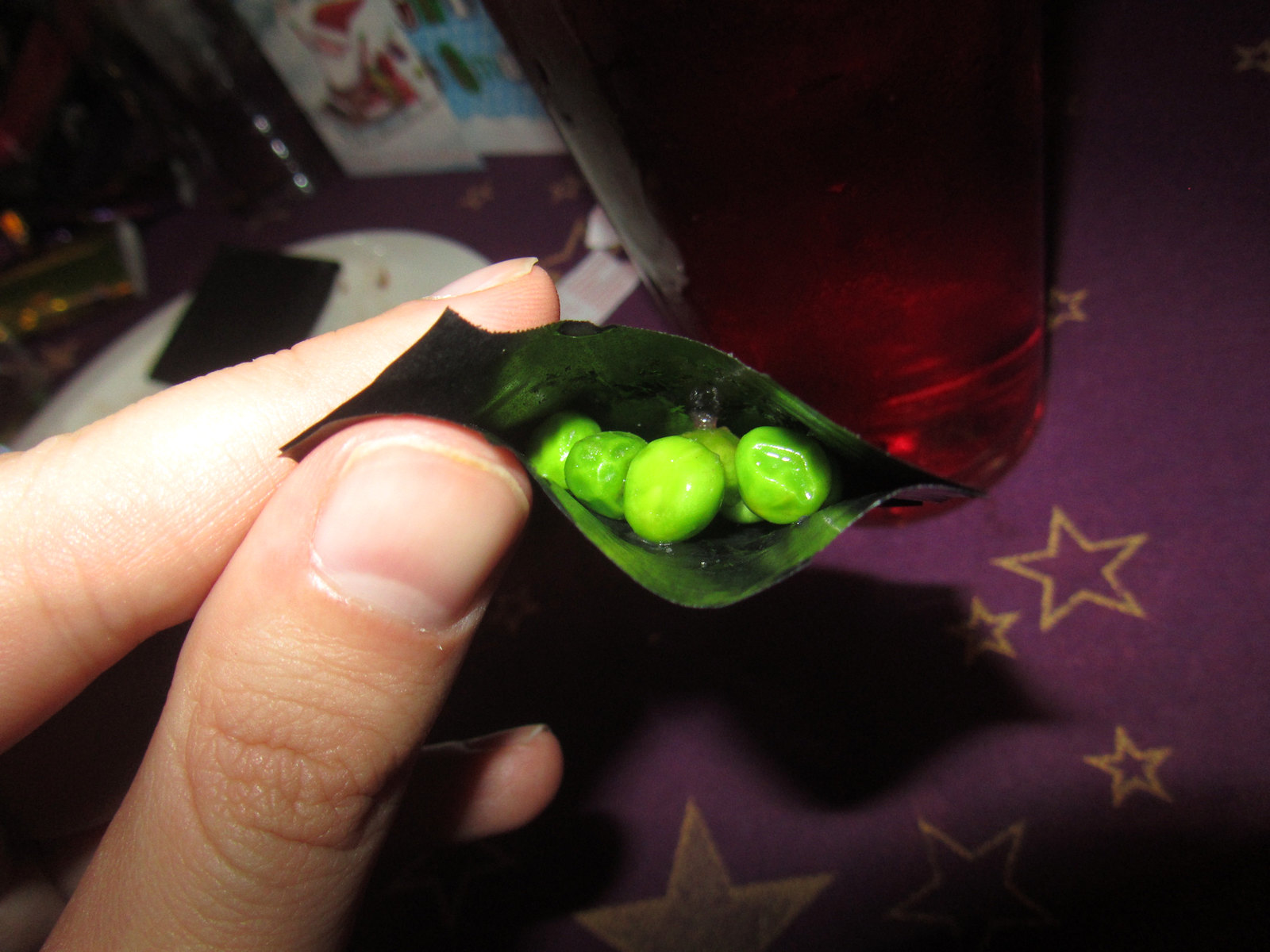In this color photograph, a white-skinned hand is holding a small foil package of bright green garden peas, potentially wasabi-flavored, against a purple tablecloth adorned with five-pointed yellow and dark grey stars. The thumb and index finger are visible, suggesting the package is being held up for display. Behind the package, there's a red drinking glass, which may actually contain a red liquid. The background includes some plates and slightly out-of-focus elements, such as what appears to be a black napkin or object on the table, and Christmas cards featuring Santa Claus, enhancing the festive ambiance. The vivid green peas inside the foil package take center stage, contrasting sharply with the richly decorated purple tablecloth.